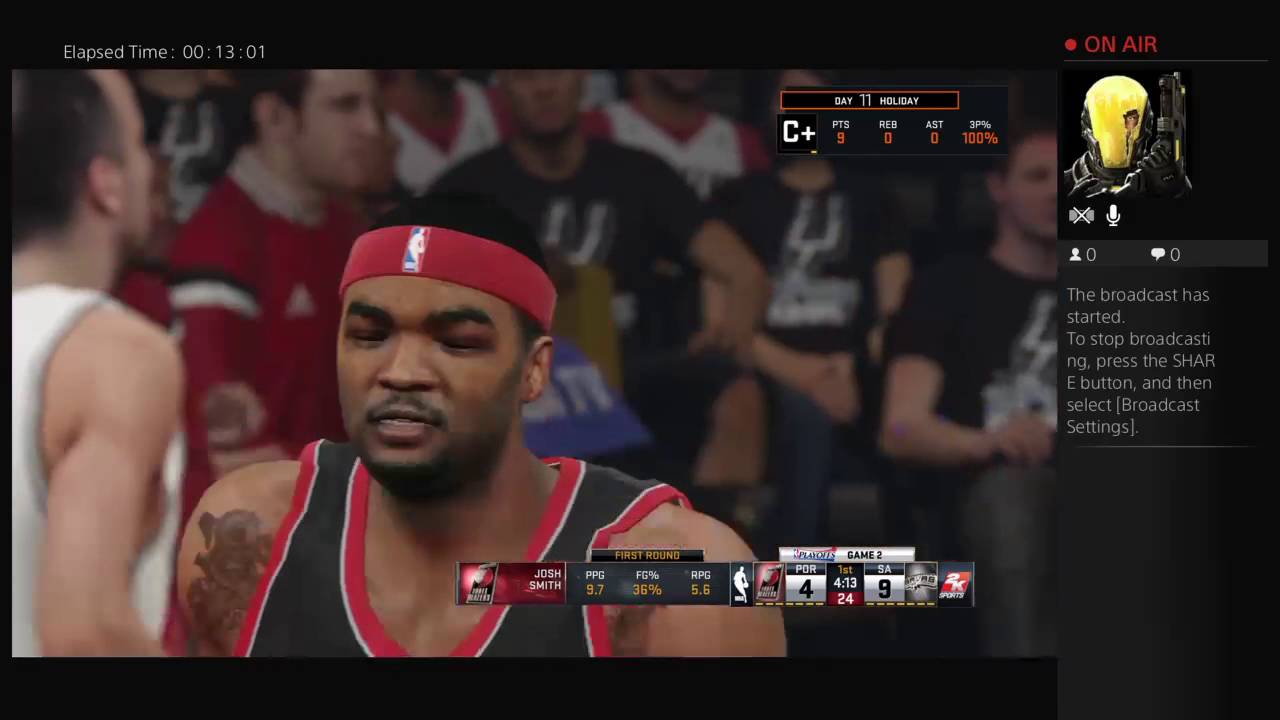A live stream showcases an intense NBA 2K video game match between the Portland Trail Blazers and the San Antonio Spurs during the first quarter, with 13 minutes elapsed. The streamer, energetically engaging their audience, highlights the growing trend of watching others play video games, which has garnered a dedicated fanbase. This modern pastime, facilitated by platforms like Twitch, allows viewers to experience the excitement of virtual gameplay vicariously, similar to social gaming gatherings of the past. However, opinions on this trend remain polarized, with some critics dismissing it as an unappealing and unproductive hobby.